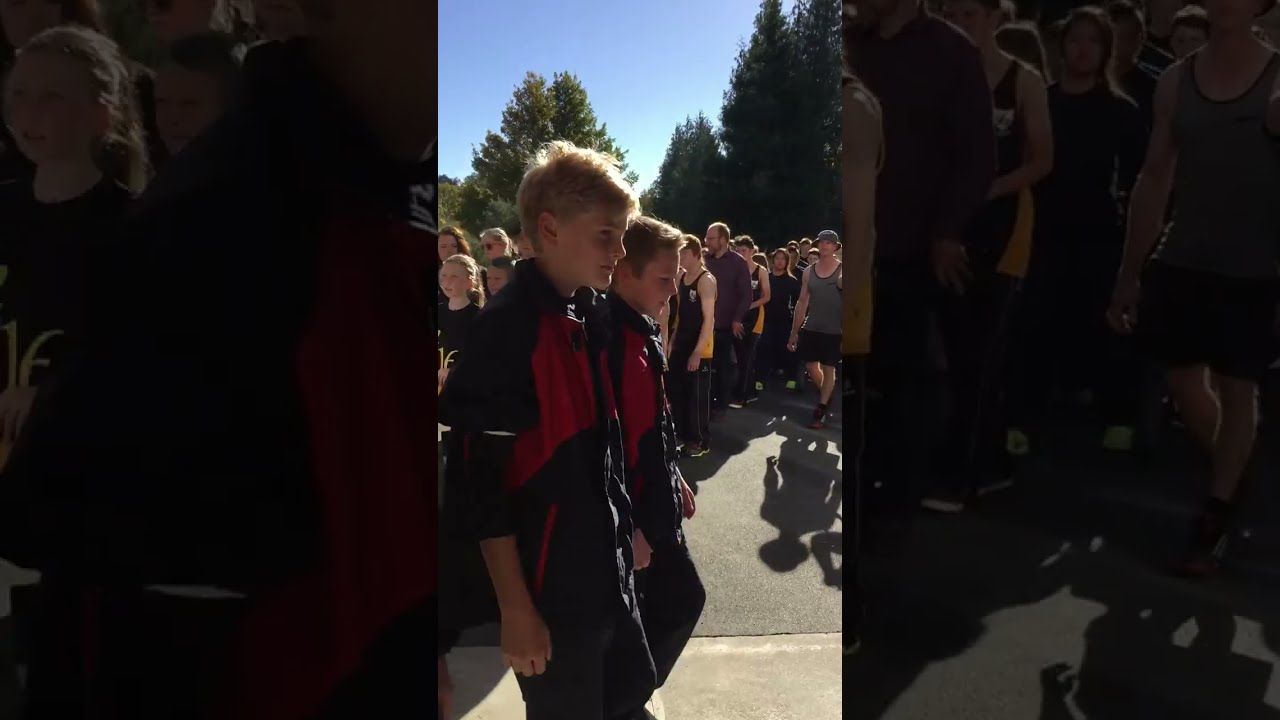In the center of the image, two young boys with blonde hair are prominently featured, both wearing identical black and red jackets, their sleeves possibly pushed up to their elbows, along with dark-colored pants. They are walking towards the right side of the image, offering a profile view. The scene appears to be outdoors during the daytime, illustrated by the blue skies and the presence of pine trees in the background. Surrounding the boys, a diverse assembly of people, including children, men, and women, are standing in line, seemingly waiting for something. Among these individuals, a man in a black tank top, black pants, and black shoes stands out, as well as another person in a long-sleeve brown shirt with balding hair and glasses. The majority of the crowd, which includes younger children in black shirts featuring a symbol and adults in casual attire such as shorts and t-shirts with hats, is focused in the same direction, creating a sense of anticipation or orderly progression. The gathering takes place on a concrete or tar surface, suggesting a ceremonial or organized event.